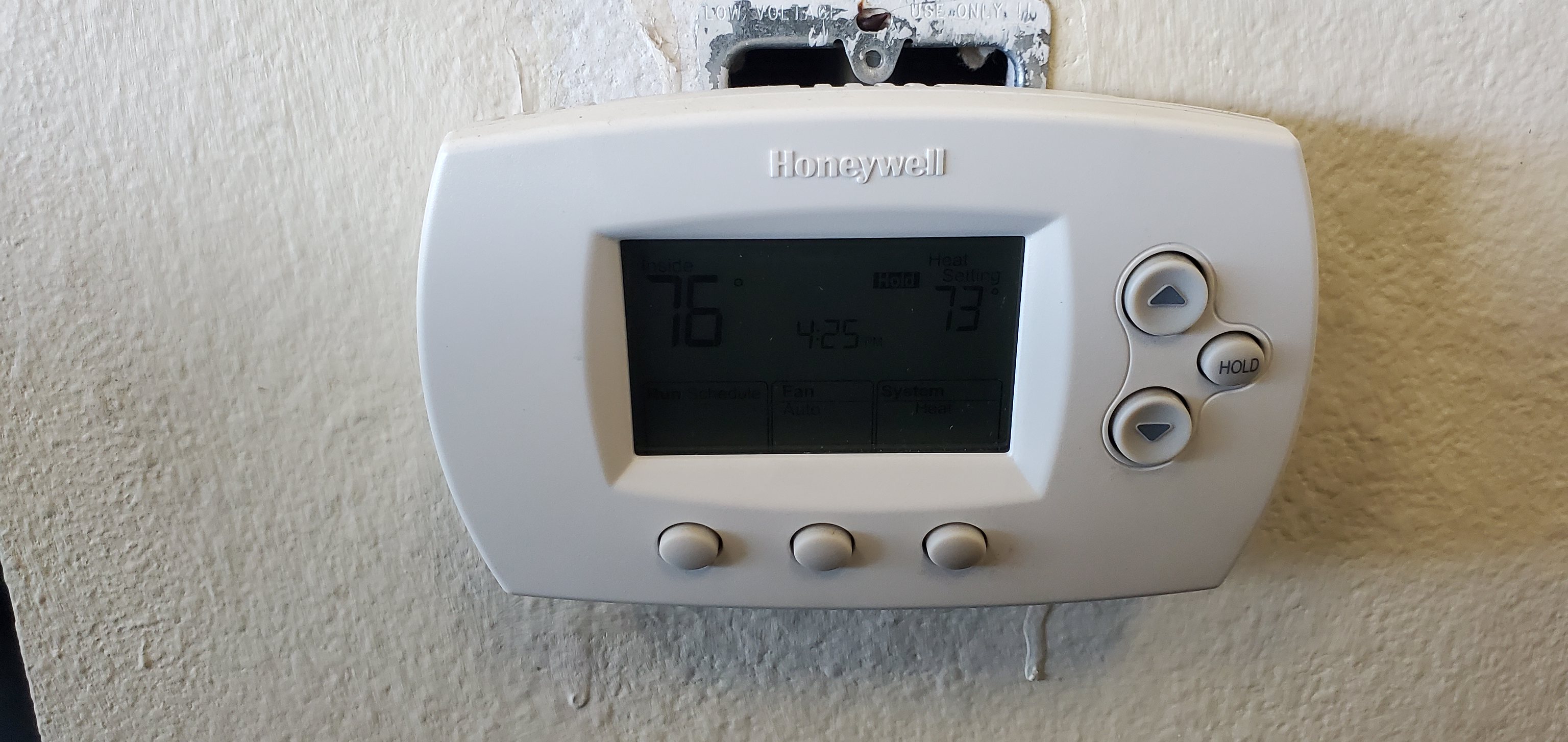A detailed color photograph captures a digital Honeywell thermostat mounted on an interior wall. The thermostat features a slightly arched, oblong design with a curved top, bottom, and sides. It includes an interactive digital display at its center, flanked by an up arrow, down arrow, and hold button for adjusting heating and cooling settings. Along the bottom are three additional buttons, although their labels are not visible.

The display currently shows a temperature of 76 degrees on the left, a time of 4:25 (AM or PM is unclear) in the center, and 73 degrees on the right. The thermostat is mounted over a vertical electrical box that is visible above and below the device, revealing a shoddy installation. The wall itself has a highly textured surface with noticeable paint drips, contributing to the overall impression of a rushed and unprofessional job. The electrical box appears old and metallic, though it might be a gray plastic one splattered with paint.